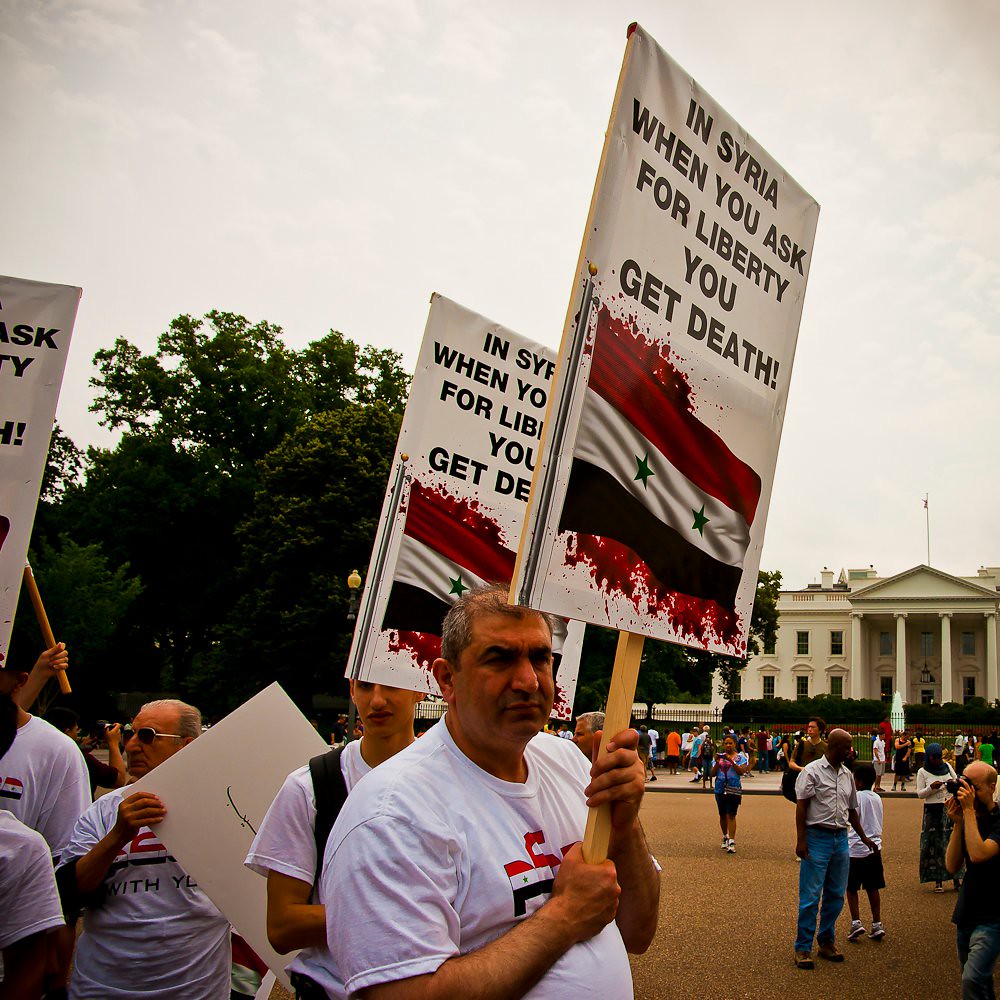The image depicts a demonstration in front of the White House on a cloudy day, where a large crowd has gathered. At the forefront, an older man in his early 60s with grayish hair stands holding a sign that reads, "In Syria, when you ask for liberty, you get death." The sign also features a Syrian flag, with red, white, and a dark color, and two stars that appear to be bleeding. He wears a white t-shirt with a logo on it. Behind him, a younger man, likely in his 20s, holds a similar sign. Another man, possibly in his 50s, stands further back holding a white sign with a line on it, looking off-screen. The overall scene is very dynamic with many people, mostly males, holding signs and moving around. The background shows the White House, some trees, and various colors including red, white, black, blue, yellow, green, and tan. The atmosphere suggests a peaceful yet somber protest, captured during the daytime.